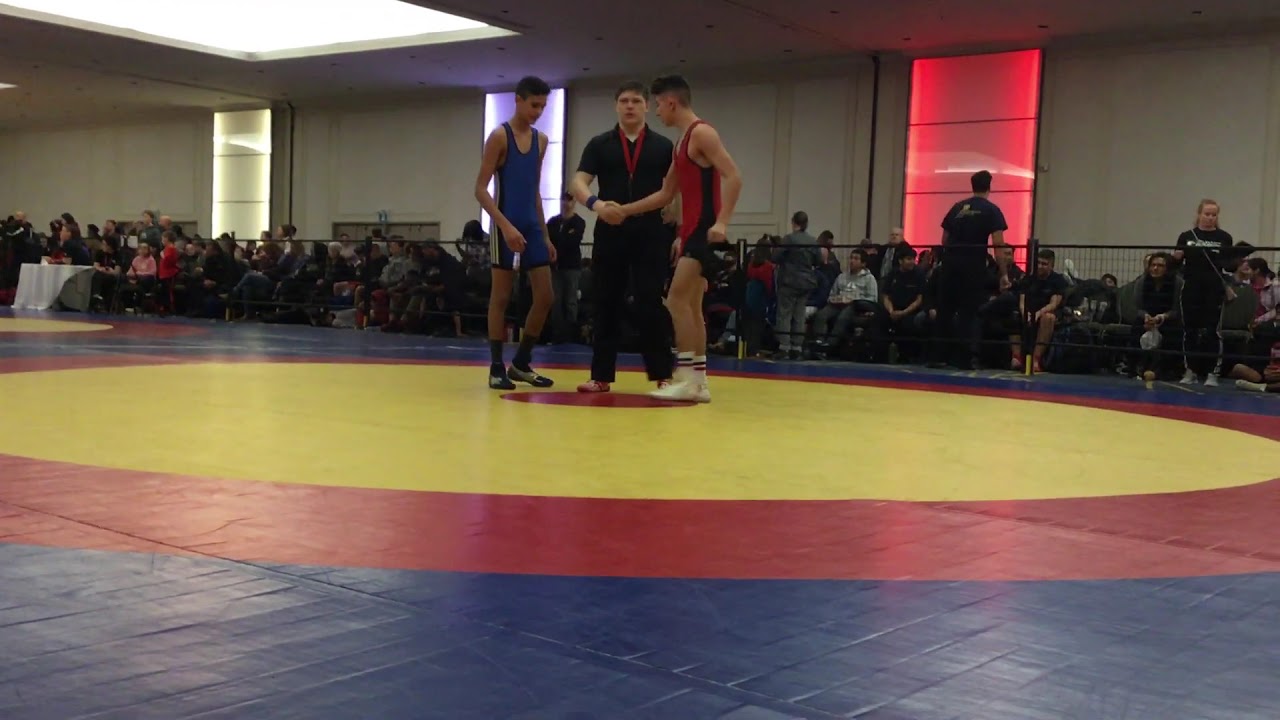The image depicts an indoor high school wrestling match in a dimly lit gym. The wrestling mat features a distinct pattern with layers of color: a blue outer edge, followed by a red ring, encompassing a large yellow circle, and a small red circle at the very center. The floor appears to be made of interlocking squares, offering a surface that balances softness and firmness for the athletes. In the center of the mat, a referee dressed in a black uniform with a red ribbon around his neck is shaking hands with the wrestler to his right, who is clad in a red and black uniform, striped socks, and white shoes. The other wrestler, donning a blue shirt and bluish-black shorts, looks down at the handshake. Behind the match, a black fence separates a seated audience from the action, providing a clear demarcation between spectators and participants. The photo is horizontally framed, capturing a moment before the wrestlers engage in their bout.